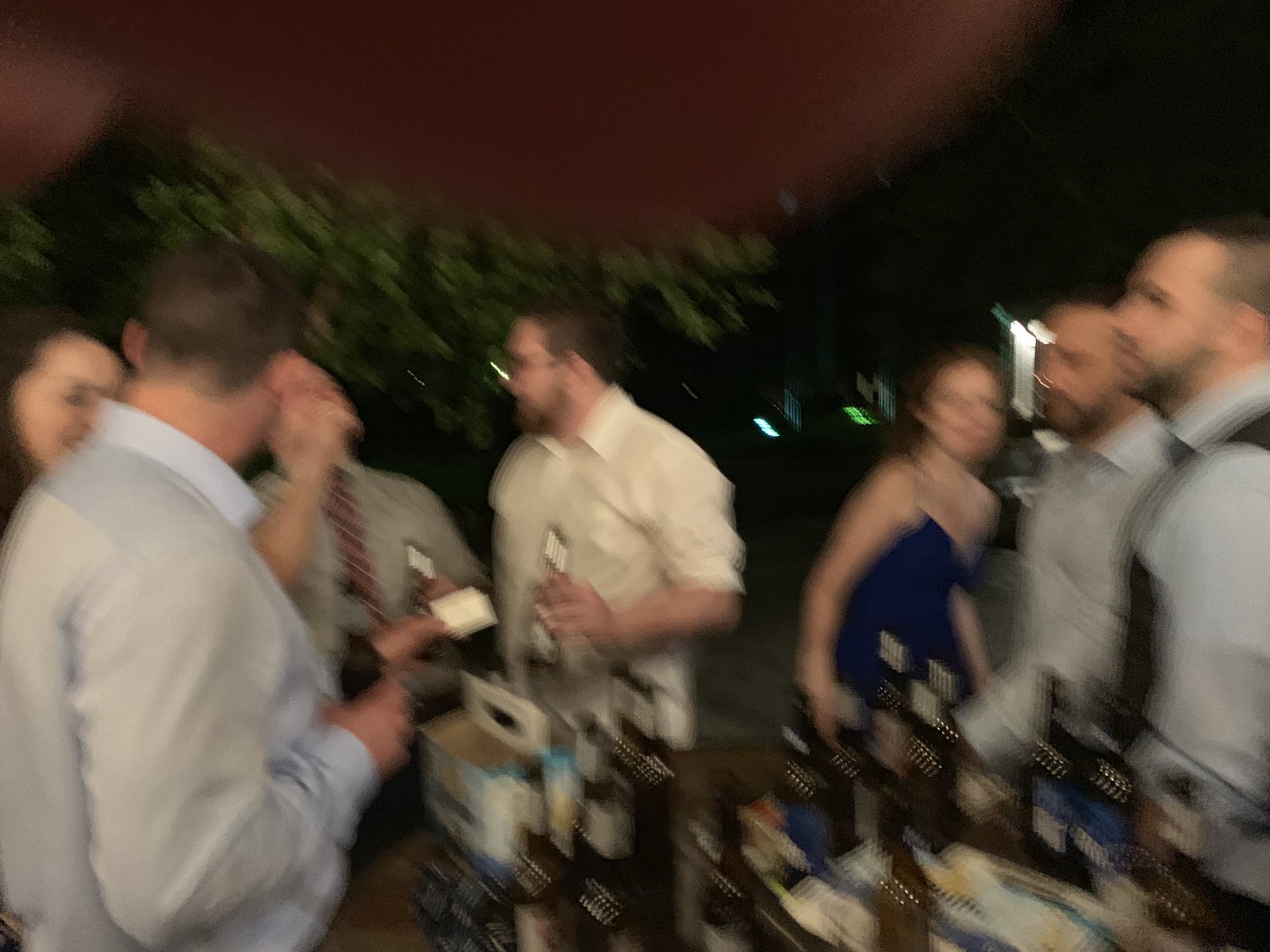This nighttime photograph captures a blurry outdoor social event, possibly a wedding reception or a dance. The upper portion of the image shows a dark sky with the faint outline of trees stretching across the background. The scene is partially obscured by the photographer's thumb in the upper corner. Gathered around a table in the foreground, seven individuals are clad in business casual and formal attire, engaging in conversation and holding beverages, predominantly beer. 

On the left side of the image, a woman in a cobalt blue spaghetti strap dress, with shoulder-length light brown hair, stands next to three men. One man in a black tie and dress shirt is chatting with two other men in dress shirts without ties, one wearing glasses and an off-white shirt with rolled-up sleeves. The men are holding beer bottles, indicating a relaxed atmosphere.

On the right side, two Caucasian men with short face stubble and balding brunette hair, both wearing gray button-up shirts—one also donning a black vest—are seen conversing. In the lower right foreground, a table is visible stocked with several brown beer bottles and their accompanying white and light brown cardboard cases. A woman in a black strapless dress appears to be walking toward the right, further adding to the dynamic and social nature of the event captured in this vivid yet blurry snapshot.